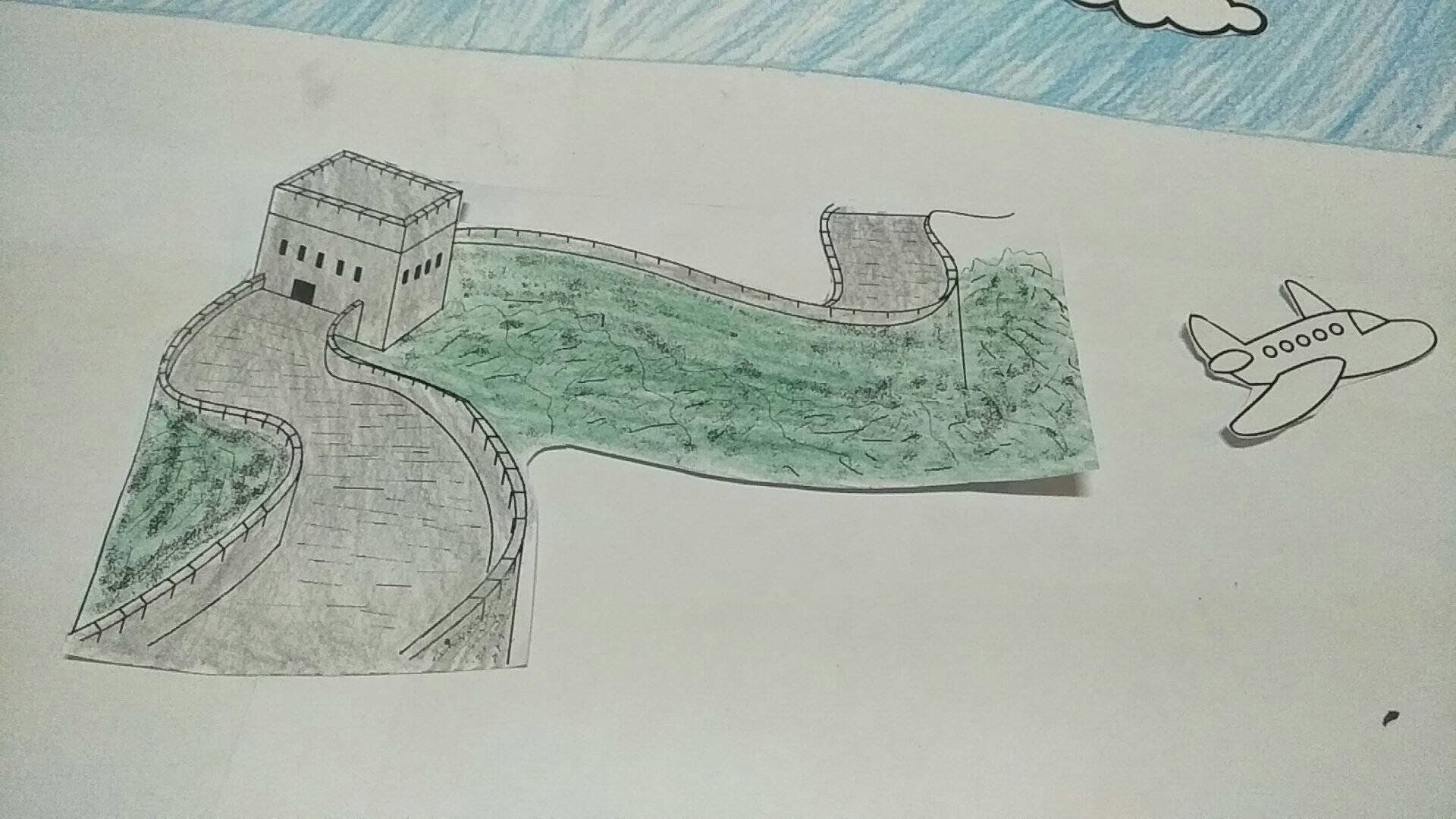This photograph captures a detailed and colorful piece of artwork, possibly created by a child. The artwork is displayed on a long, white poster board resembling a banner. At the top of the poster, there is a section shaded with blue colored pencil to represent the sky. Overlaying the sky, there's a cut-out cloud outlined in black marker. On the right side of the composition, a small, black-outlined cartoon plane has been cut out and pasted onto the poster. Dominating the left side of the artwork is an intricate depiction of the Great Wall of China. This segment appears to be cut out and pasted onto the board, with the wall itself colored in gray pencil and surrounded by green areas, likely representing the surrounding landscape or hills. The artist has made an effort to include perspective, showing the wall snaking around a hill and including a notable structure within the wall, enhancing the overall depth and realism of the scene.